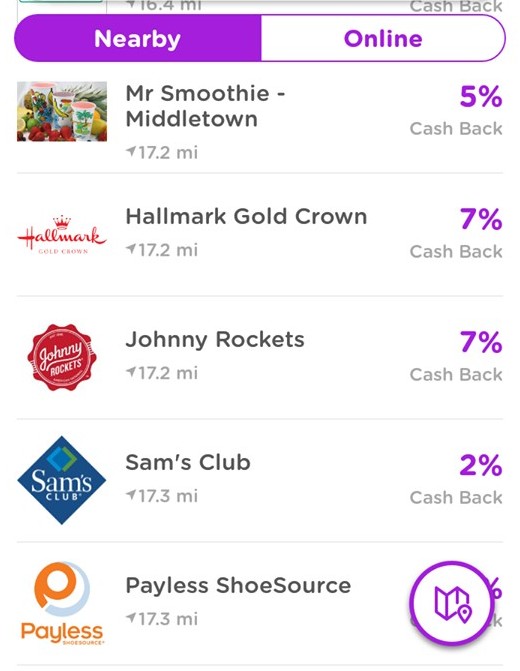Screenshot features a complex cash back display interface. At the top left, it shows "16.4 miles," and on the top right, it says "Cash Back." Below, there is a purple button labeled "Nearby" in white letters and a white button labeled "Online" in purple letters. The main content area includes images and details of various offers:

1. A picture of three smoothies in cups, surrounded by fruits in the background, with the text "Mr. Smoothie, Middletown, 17.2 miles, 5% cash back."
2. The Hallmark Gold Crown icon accompanied by the text "Hallmark Gold Crown, 17.2 miles, 7% cash back."
3. The Johnny Rockets logo with the text "Johnny Rockets, 17.2 miles, 7% cash back."
4. The Sam's Club logo followed by the text "Sam's Club, 17.3 miles, 2% cash back."
5. The Payless Shoes logo is also present, suggesting more deals available.